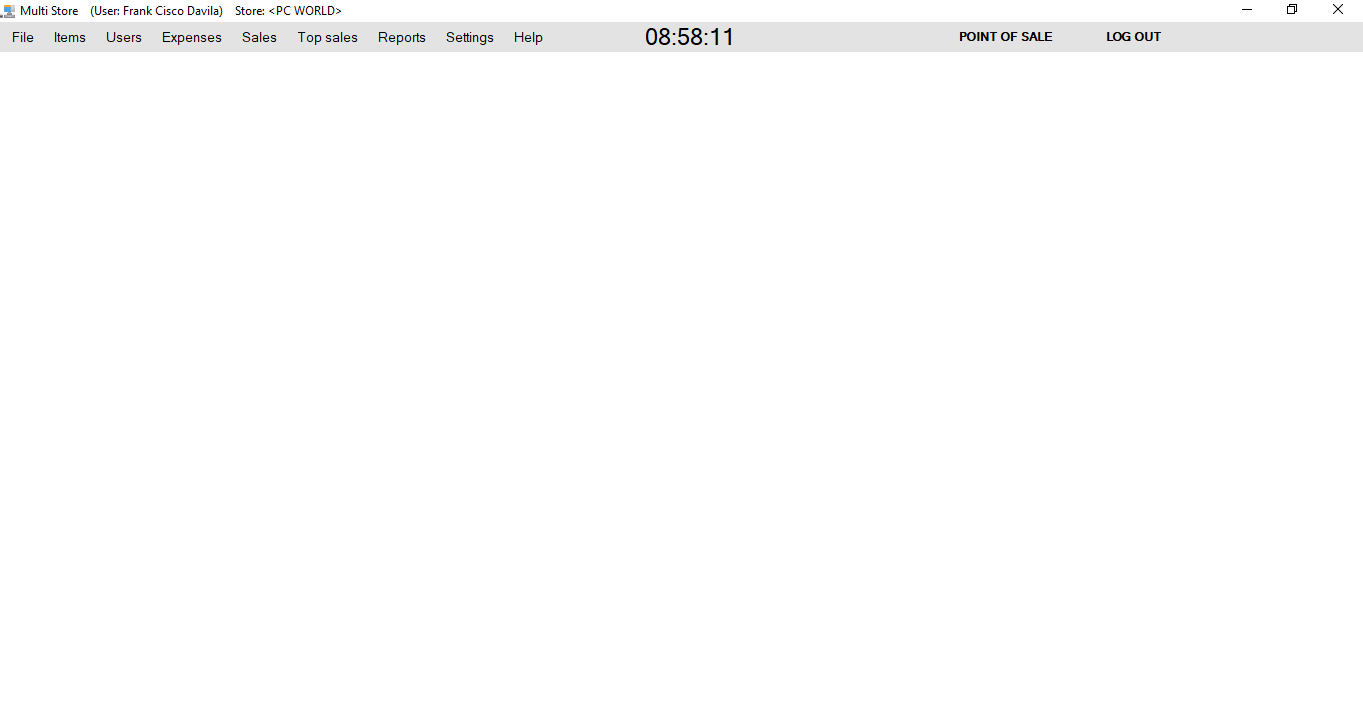This screenshot captures a minimalist software interface primarily dominated by a white background. The interface features two header bars at the top.

The first header bar has a white background and starts on the upper left with a small computer icon rendered in gray, adorned with small blue and orange accents. Following this icon is the text "MULTISTORE," immediately succeeded by "(USER FRANK CISCO DEVILLE)." To the right of this, it states "STORE: <PC WORLD>" in uppercase letters. A significant gap of white space stretches across the middle of this bar, culminating on the far right with three web navigation icons: a horizontal line to minimize, an icon depicting overlapping squares to represent multiple pages, and a gray 'X' to close the page.

Beneath this is a smaller gray header bar featuring various drop-down menu options on its left side. These options include "File," "Items," "Users," "Expenses," "Sales," "Top Sales," "Reports," "Settings," and "Help." Centrally on this gray bar, in a slightly larger and bolder black font, is the time displayed as "08:58:11." Towards the right, but not fully aligned to the edge, are the bold, uppercase texts "POINT OF SALE" and "LOGOUT."

The central area of the page below these headers remains largely white, with the two header bars occupying only a small fraction at the top.